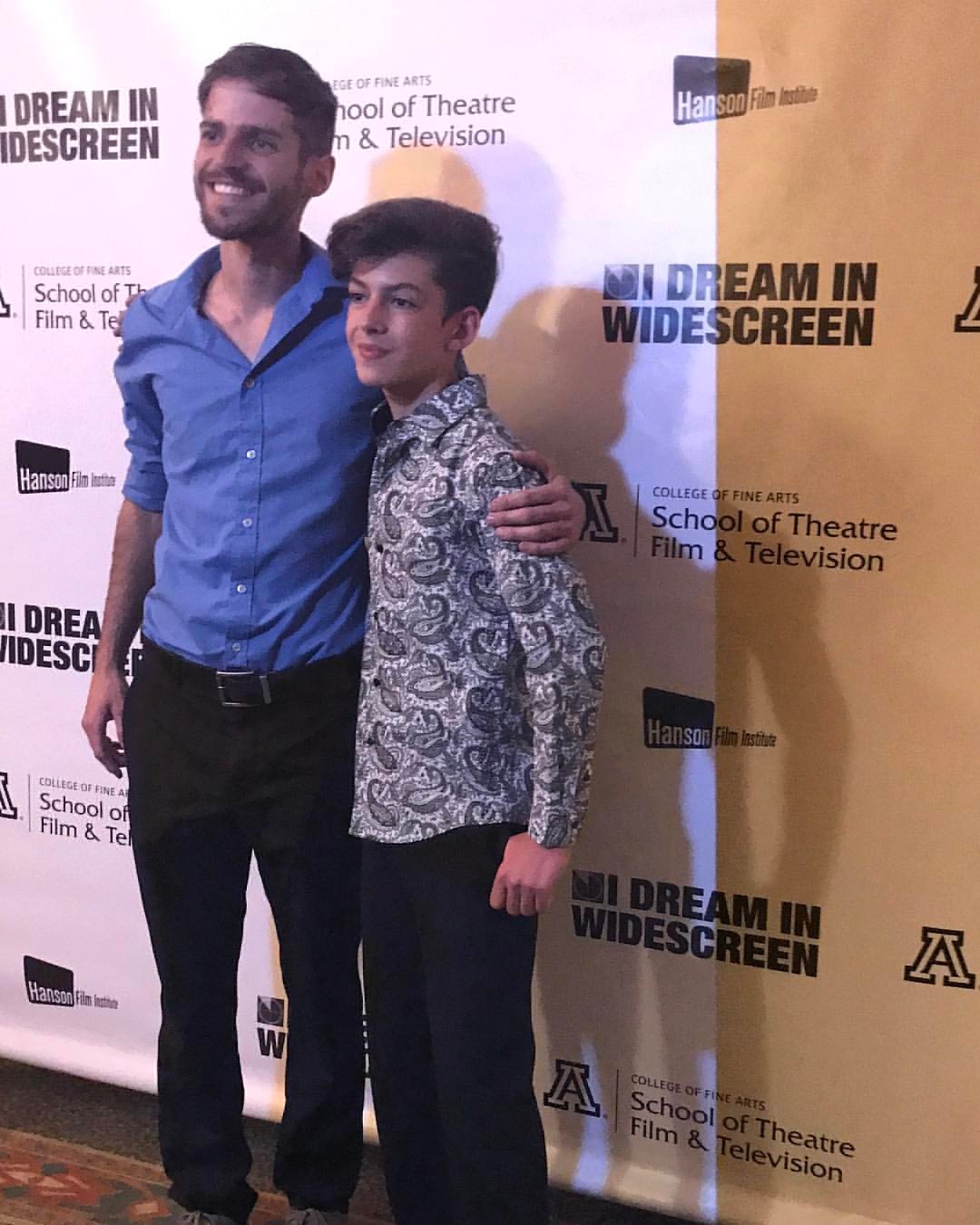In this captivating image, a man and a young boy stand arm-in-arm in front of a professional backdrop. The man, dressed in a blue button-up shirt, black belt, and black pants, has his arm affectionately wrapped around the boy's shoulder. The boy, sporting black pants and a gray and white shirt with intriguing designs, smirks subtly while the man beams a warm smile. Both are gazing off to the left, suggesting their attention is focused on a different camera than the one capturing this moment. The white backdrop behind them prominently features repeated black ink text that reads, "I Dream in Widescreen," alongside the logos for the College of Fine Arts at the University of Arizona, the School of Theatre, Film, and Television, and the Hanson Film Institute. Their shadows are clearly visible on the backdrop, adding depth to the scene.